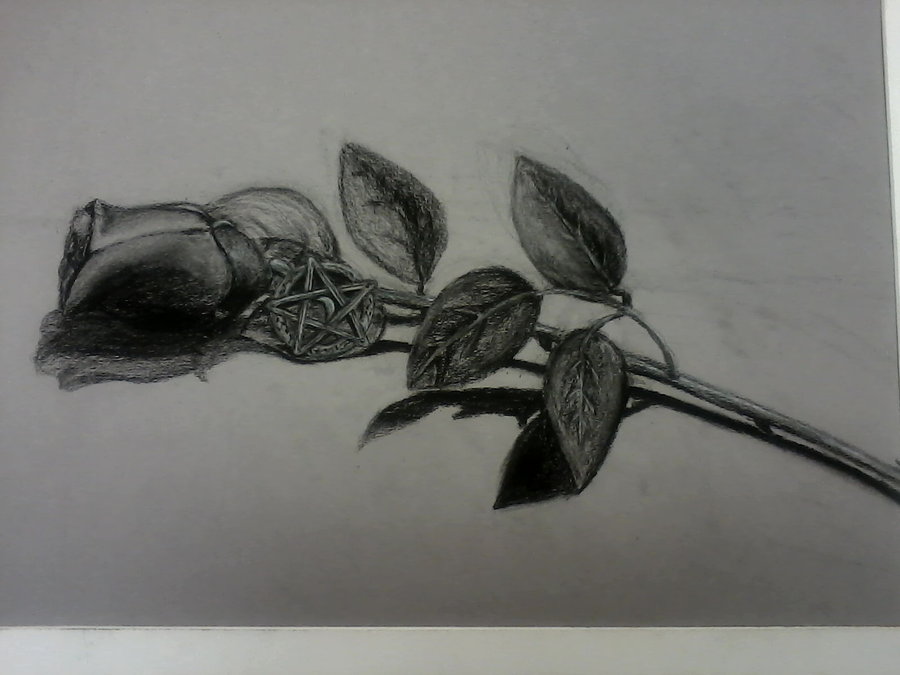The image features a meticulously crafted charcoal drawing of a single, long-stemmed red rose. The rose's head gracefully points to the left, while its stem extends diagonally across the picture towards the right. Adorning the rose's bud is a necklace made of cloth, intricately wrapped around it. This necklace includes a pentagram charm, which is circular in shape and contains a Star of David design with an additional circle at its center. The pentagram is rendered in an off-grayish tone, providing a striking contrast against the rose. The rose itself is detailed with five distinct petals unfurled from its bud. The backdrop of the artwork features a nuanced blend of off-white and dark-gray shades, adding depth and texture to the overall composition.